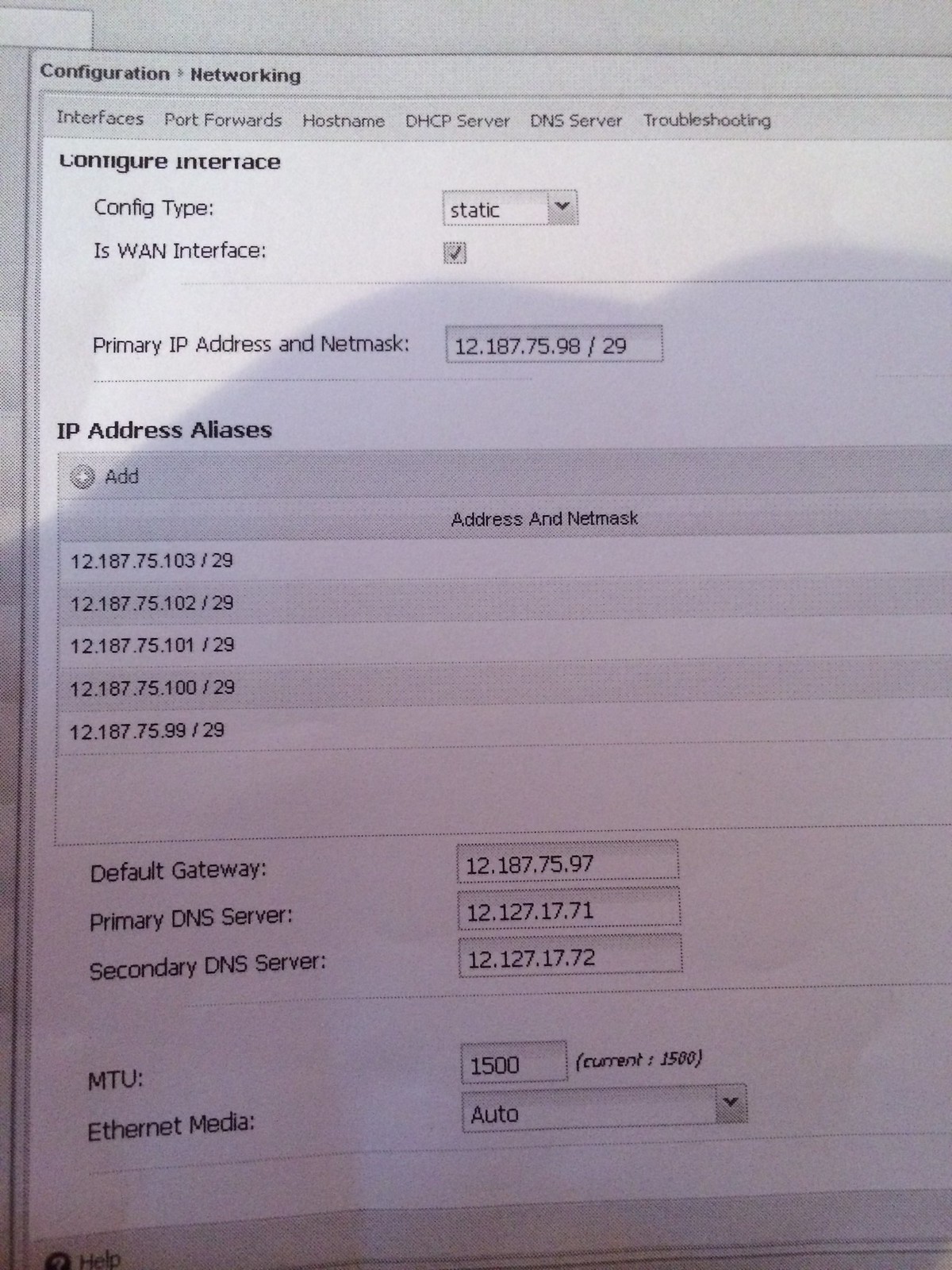The image is a black-and-white photograph of a computer screen displaying a detailed networking configuration interface. The predominant background color is pale gray with black lettering. The interface is titled "Configuration Networking" and includes numerous text fields and options related to network settings. Key sections and elements visible in the image include:

- **Interfaces**: Lists various networking elements such as "port forward," "hostname," "DHCP server," "DNS server," and "troubleshooting."
- **Primary IP Address and Netmask**
- **Default Gateway**: Shows the current default gateway IP address.
- **Primary and Secondary DNS Servers**: Provides fields for the primary and secondary DNS server addresses.
- **Ethernet Media**: Has a drop-down menu with "auto" selected.
- **Configure Interface**: Offers options to set configuration type, with "static" and "WAN interface" being notable settings that are checked.

The interface is designed for advanced network configuration, allowing users to modify settings related to IP addresses, netmask, DNS servers, and other network parameters. The shadow on the image suggests it is a photograph of the screen rather than a direct screenshot.